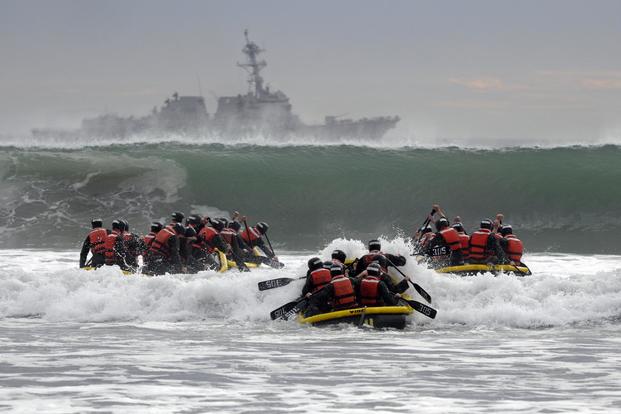In this dynamic image, we observe five black and yellow boats, each filled with more than six military trainees, likely undergoing Navy SEAL training. The trainees are uniformly equipped with red life jackets, black helmets adorned with a white identifying strip, black shirts, and black pants. Each one grips a black paddle as they navigate through the tumultuous gray waves of the ocean. The scene captures them paddling determinedly through the heavy surf toward an imposing, large wave that dominates the middle of the image. In the background, beyond the crashing waves, a mammoth Navy ship equipped with a formidable front gun and missile launchers stands sentinel. The somber, overcast skies and the dark, choppy ocean add a layer of intensity and challenge to their rigorous training session.